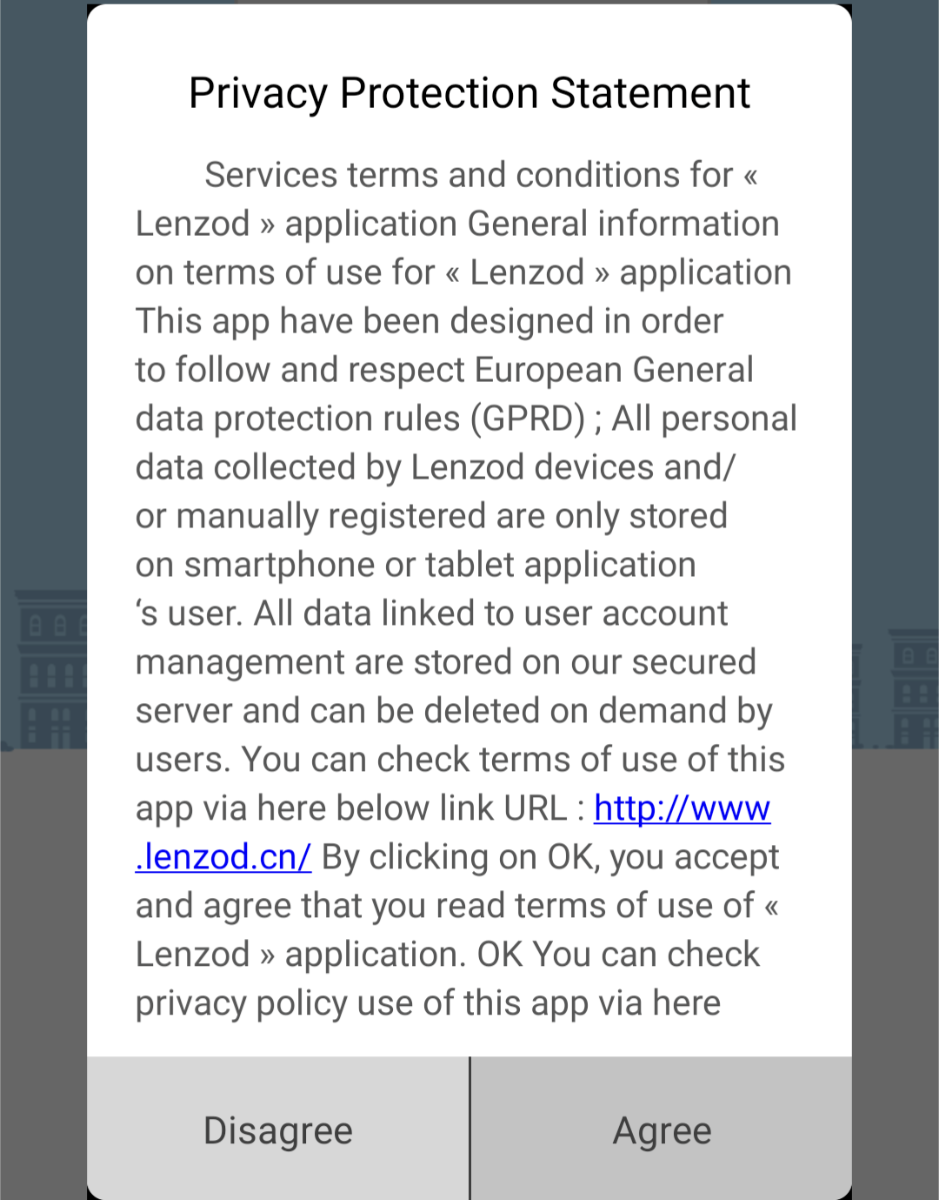This image is a mobile screenshot displaying a privacy protection statement for the company LensOdd. The image is tall and rectangular, lacking a top bar, and features a pair of buttons that are consistent with mobile device interfaces. The text at the top clearly states that this is a "Privacy Protection Statement," followed by a detailed block of text outlining the terms and conditions of use for the LensOdd application.

At the bottom of the statement, there are two buttons: "Disagree" located in the bottom left corner and "Agree" in the bottom right corner. The "Agree" button is slightly grayed out, indicating that it is currently being pressed. This screenshot appears to have been captured at the moment the user is interacting with the "Agree" button.

The text explains that the LensOdd app complies with European General Data Protection Regulation (GDPR) standards. It emphasizes that all personal data collected by LensOdd devices, whether automatically or manually, are stored exclusively on the user's smartphone or tablet. Data related to user account management is securely stored on LensOdd's servers and can be deleted upon user request. The statement also acknowledges minor typos within the text.

For further details, users are directed to the terms of use and privacy policy, accessible via a provided URL: http://www.lensodd.cn. The user must click "Okay" to confirm that they have read and agreed to the terms and conditions outlined in the statement.